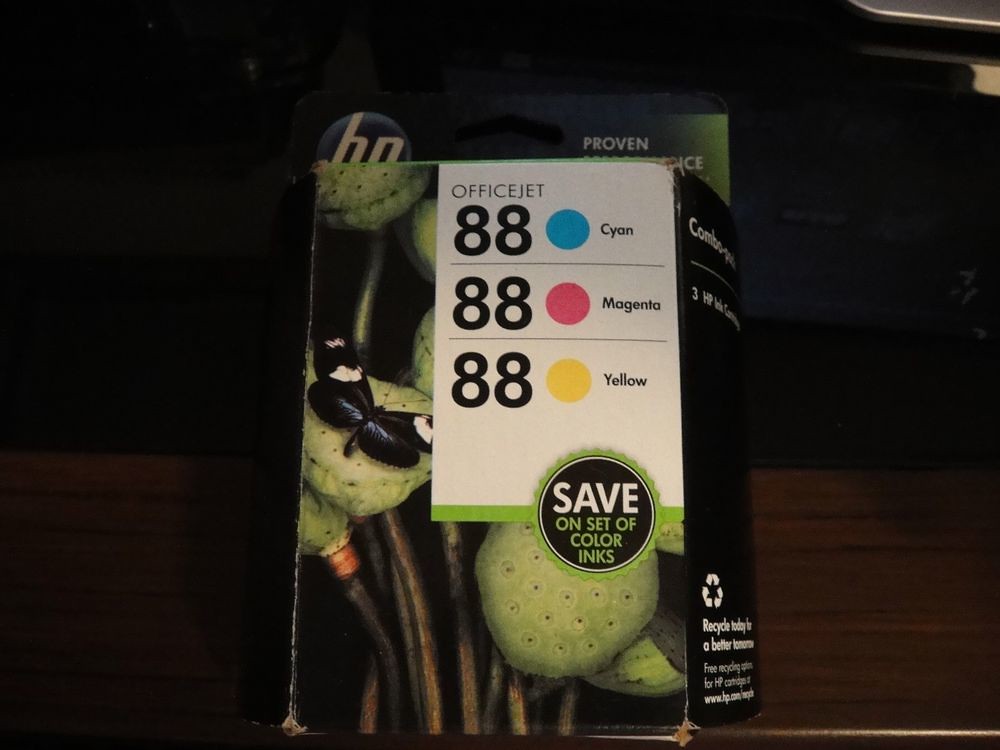The photo depicts an HP-branded cardboard box resting on a dark wooden surface, which looks like a table or desk. The box is slightly worn, with visible wear on its corners. The front of the box features a prominent white label with the word "OfficeJet" at the top, followed by the numbers "88" in three places, each accompanied by a colored dot—blue for cyan, pink for magenta, and yellow for yellow. The label also includes the text "save on set of color inks." There's a recycling logo at the bottom right of the package. The background of the packaging showcases green plant seed pods, possibly poppy pods, and a black and white butterfly. One side of the box is slightly pushed out, revealing more details about recycling.